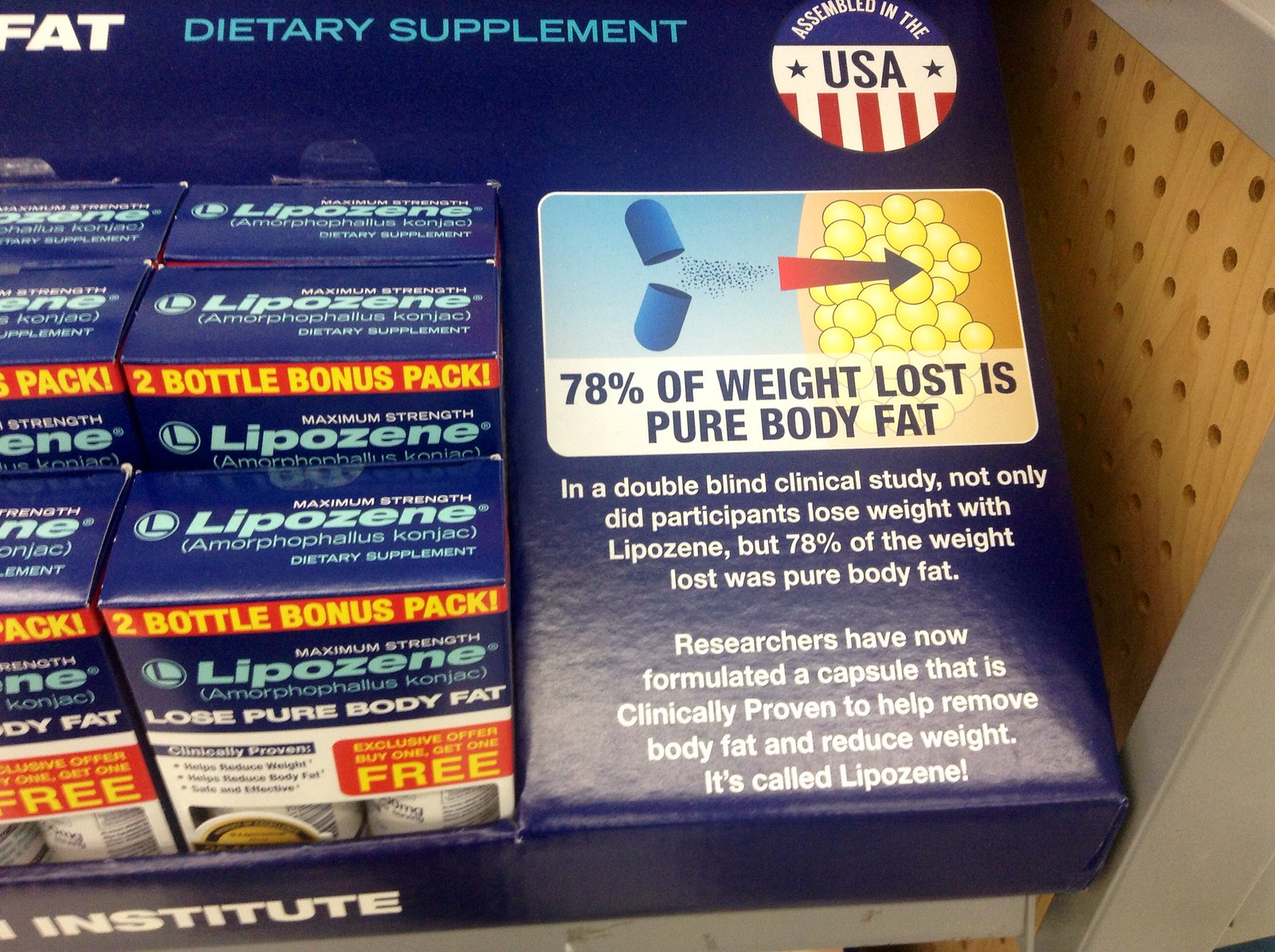The image captures a neatly organized retail shelf inside a store. The shelf frame is gray and features wooden pegboard siding for a sturdy, yet utilitarian look. Prominently displayed on the shelf is a large blue display box containing several smaller boxes of Lipozene, a dietary supplement designed for weight loss. Each small box houses two bottles of the supplement. The packaging highlights noteworthy claims such as "78% of weight loss is pure body fat," based on the findings of a double-blind clinical study. The text also emphasizes that not only did participants lose weight with Lipozene, but a significant portion of the weight loss was specifically body fat. The researchers behind Lipozene have developed capsules that are clinically proven to assist in fat removal and weight reduction. The display is attractively arranged to catch the eye of potential customers seeking weight loss solutions.